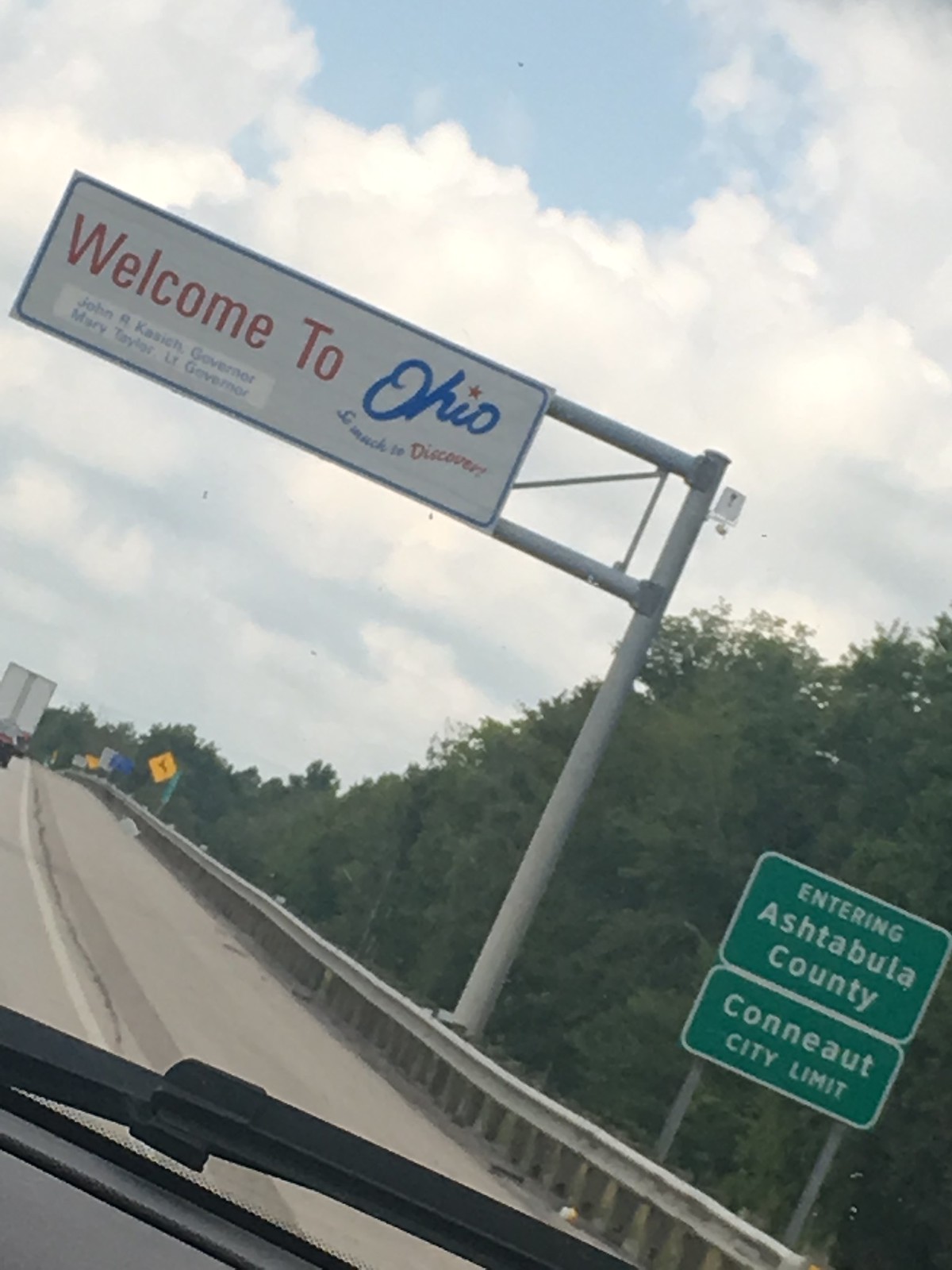This photograph, taken from the right lane of an interstate, captures a vibrant moment on the road. The car's windshield washers and wipers are faintly visible at the edges of the frame, adding a touch of realism. Looming above, a prominent sign proudly declares: "Welcome to Ohio - So Much to Discover." Flanking this sign are two smaller green signs, one indicating entry into Ashtabula County and the other marking the Canoe City limits. In the distance, a yellow deer crossing sign alerts drivers to potential wildlife. Metal guardrails line the highway, providing safety and structure, while a lush canopy of green trees envelops the scene, offering a serene backdrop to this portion of the journey.